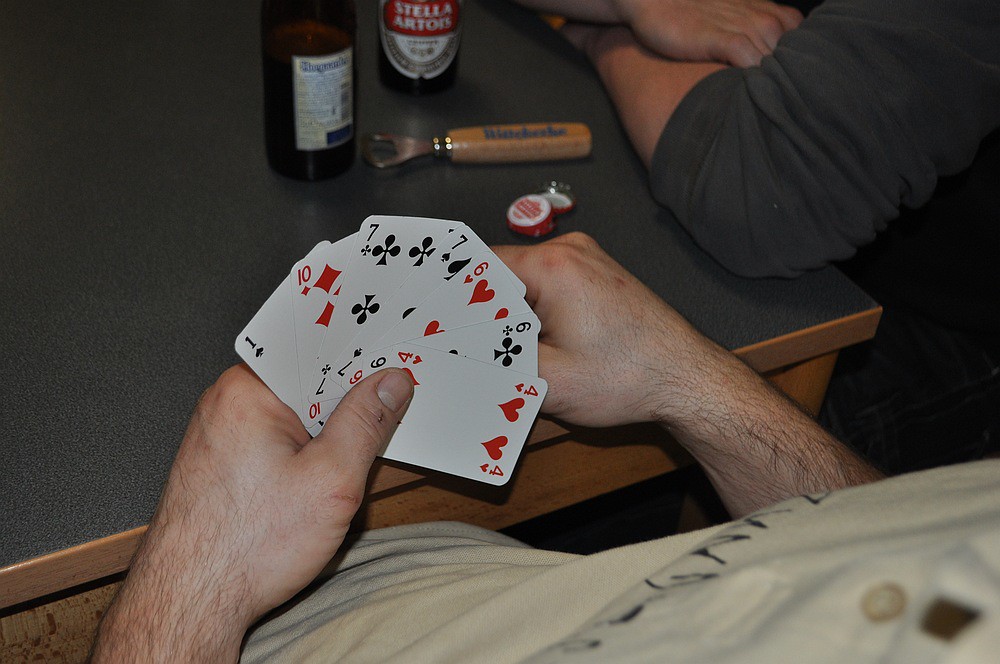In this photograph, a young gentleman is immersed in a game of cards, holding a hand that appears to be moderately good. Positioned to his right, another man with folded arms rests them on the table, indicating he may not be participating in the game. The setting suggests a casual, intimate ambiance, as evidenced by two bottles of beer on the black tabletop—one clearly labeled Stella, while the other remains turned away, its label out of view. Scattered bottle caps and a bottle opener further enhance the laid-back atmosphere. The table itself features a sleek black surface atop a woodgrain base, adding a touch of rustic charm to the scene.